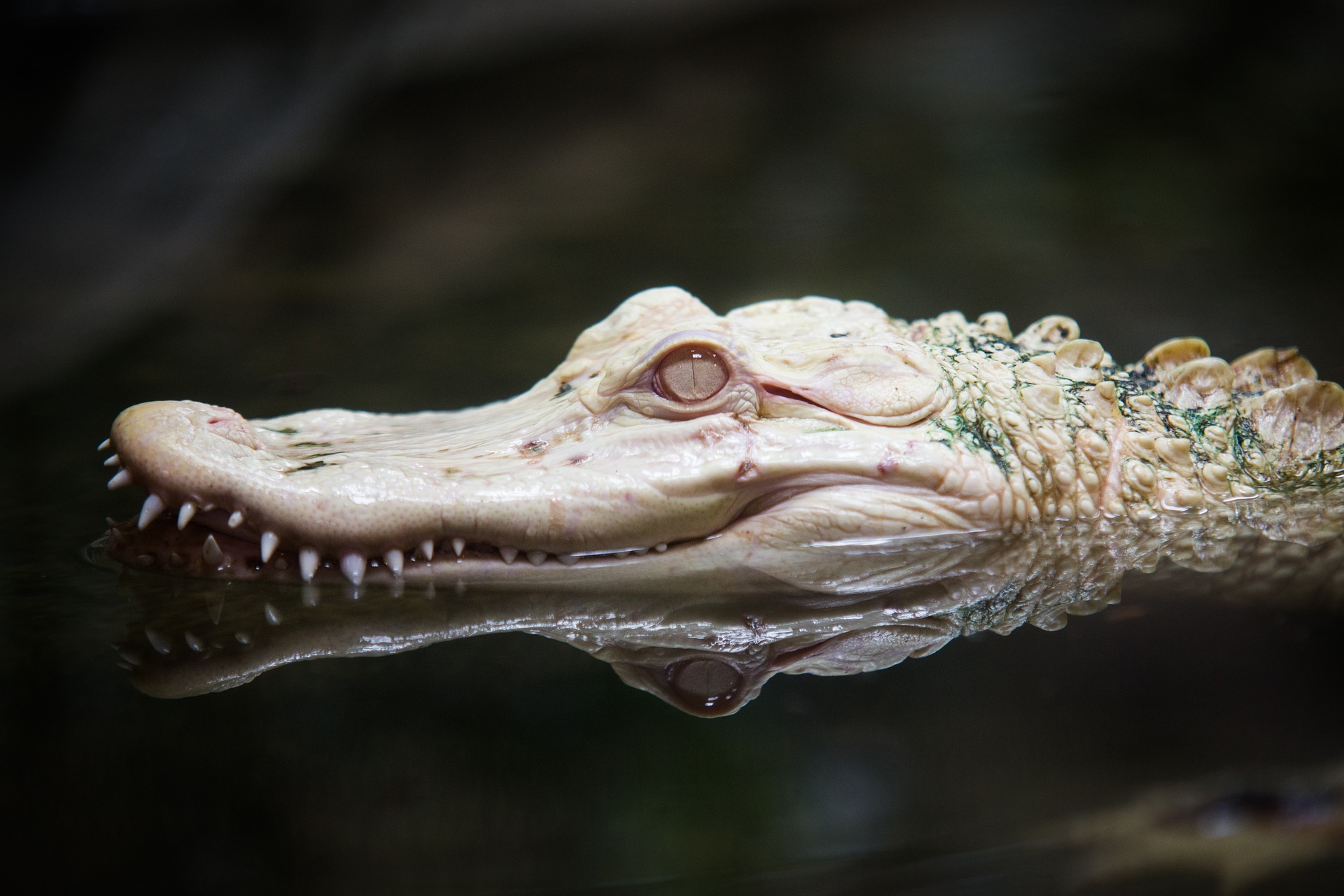The image features an albino crocodile or alligator, identifiable by its long mouth and slightly open upper jaw lined with sharp teeth. Its body and top jaw are a creamy white color, while its eyes, which have a vertical slit pupil, exhibit a reddish or tan tint. Dark green moss or algae appears on its rough-scaled back and neck, giving it a somewhat mossy appearance. The alligator or crocodile is depicted floating in dark water, with a clear reflection of its form beneath it. The overall background is dark, enhancing the visibility of the creature's pale, almost unrealistically perfect skin. Spikes protrude from its back, intermingled with brown and cream-colored markings that resemble half-moon shapes or mushrooms. The water, filled with subtle swirls, provides a dramatic contrast to the lighter tones of the animal, reinforcing its albino characteristic and the surreal quality of the scene.